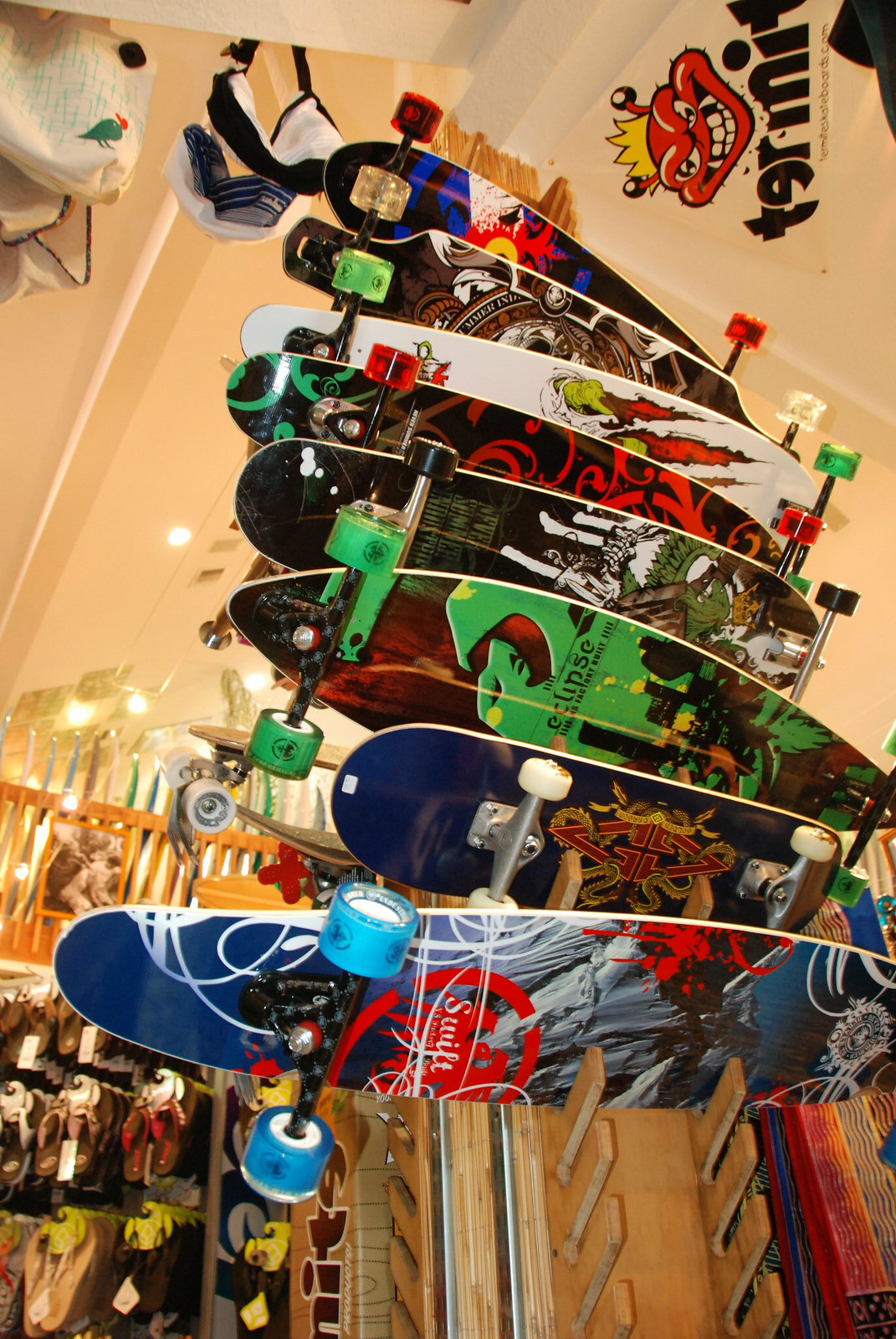This photograph, taken in color and portrait format, depicts a display of eight skateboards stacked vertically on a wooden rack inside a skate shop with a high, two-story ceiling. Each skateboard showcases a unique design and colored wheels, emphasizing their individuality. Starting from the front, the first skateboard has a round edge, blue wheels, and blue and silver artistry on its underside. The next is a shorter skateboard with rounded edges, white wheels, and a bluish background featuring a red and gold image. Behind it, a skateboard with lime green wheels and thinner edges stands out with a reddish and lime green background, inscribed with "Eclipse." Another skateboard features black wheels, a black background, and white and green patterns. The remaining skateboards are partially obscured but contribute to the vibrant display. To the top right of the image, a banner displays a red demon-like face with gritted teeth and a yellow crown, along with the word "Termite." Flip-flops are visible for sale on the bottom left of the image, adding further context to the shop setting. The entire scene is illuminated by the store's ceiling lights, adding a sense of depth and atmosphere to the space.